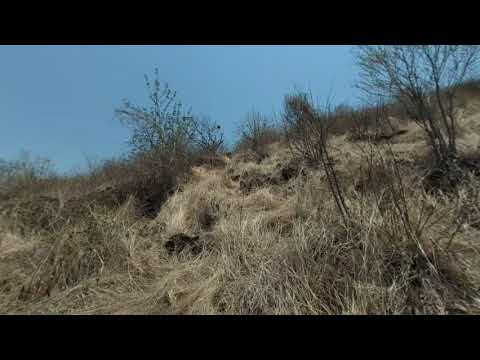The image portrays a desolate hillside dominated by dried, overgrown weedy grass that resembles hay, with sparse, dried-out trees scattered throughout the scene. The landscape, predominantly brown and tan, features brush and sticks on the ground, creating a rugged and uninviting terrain. In the midst of this barren wilderness, a small black head with ears, possibly a house cat, can be seen poking through the dry grass. The sky above is mostly a rich blue with thin, wispy clouds. The photo is framed by thin black rectangles at both the top and bottom, emphasizing the contrast between the vivid sky and the bleak, dry ground. This wide expanse of nature feels forlorn and wild, adding a sense of isolation to the image.